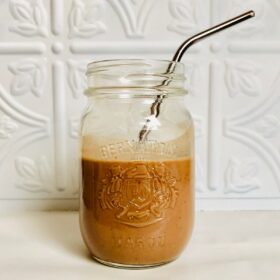A vintage-style mason jar sits on an ivory countertop, containing a two-thirds full portion of an unappealing brownish-orange liquid. The liquid leaves a visible stain about an inch above its surface. The jar, which may have once held spaghetti sauce, features a partially legible logo and text that seems to spell "Ragu" below and something like "BER..." above, possibly "Bernadellis." A metal straw protrudes from the jar to the right. The scene is set against a striking black backsplash composed of white tiles, each adorned with a square pattern featuring a center dot and a charming design of a small berry with leaves.